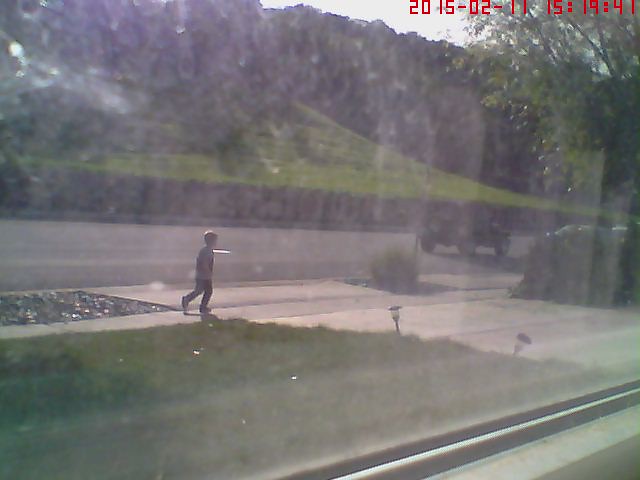The image, taken with a digital camera, has a date and time stamp in red font at the top right corner, reading "2-11-2015" at "15-19-41." The photo appears to be shot from inside looking out through a slightly dirty and streaky window, featuring a white windowsill. Outside, the scene captures a front yard with neatly trimmed green grass and two slightly leaning solar lamps. A cement walkway extends from the bottom left corner, leading to a wider driveway and a street situated on the left of the frame. 

In the middle of the image, a small boy, possibly around 6 years old with brown hair, can be seen standing near the driveway. He is dressed in dark pants and a gray shirt with some detailing on the front that isn't clearly visible. The boy appears to be looking or walking towards the street. 

To the right side of the image, a black Jeep is seen, somewhat out of focus, driving towards where the boy is standing. The background reveals a stone retaining wall with a grassy hill ascending behind it, along with several trees standing tall in the distance.